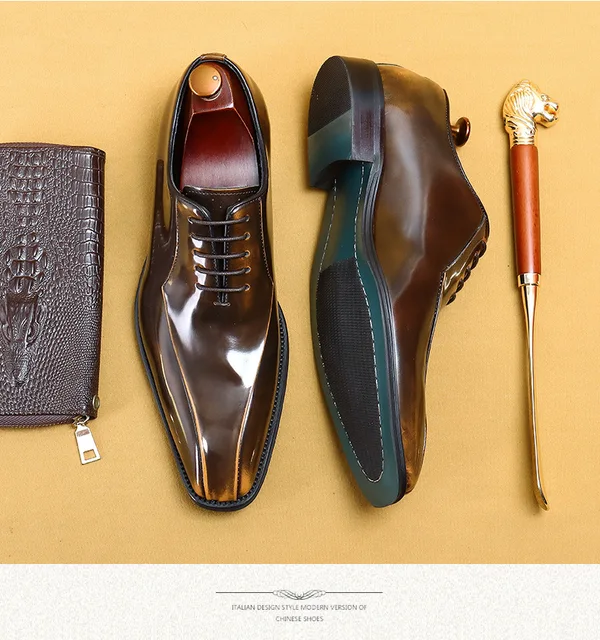The image features a meticulously arranged composition on an orange-beige background, showcasing a polished pair of dark brown leather shoes. These shoes come with dark wooden shoe stretchers inside, each topped with a gold or brass-colored knob. The shoes are highly shined, with one standing upright and the other laying on its side, exposing the stitched sole and half-inch heel. Alongside the shoes, a gold-colored shoe horn with a medium brown handle and a horse head design rests to the far right. On the far left, there's a sleek leather case embossed with a crocodile pattern and a visible white zipper, hinting at Italian design, possibly stated as "Italian design style, modern version of Chinese shoes." Also visible is a dark brownish-black leather wallet and an ornate lion-headed walking stick, suggesting an image of luxury and detailed craftsmanship.